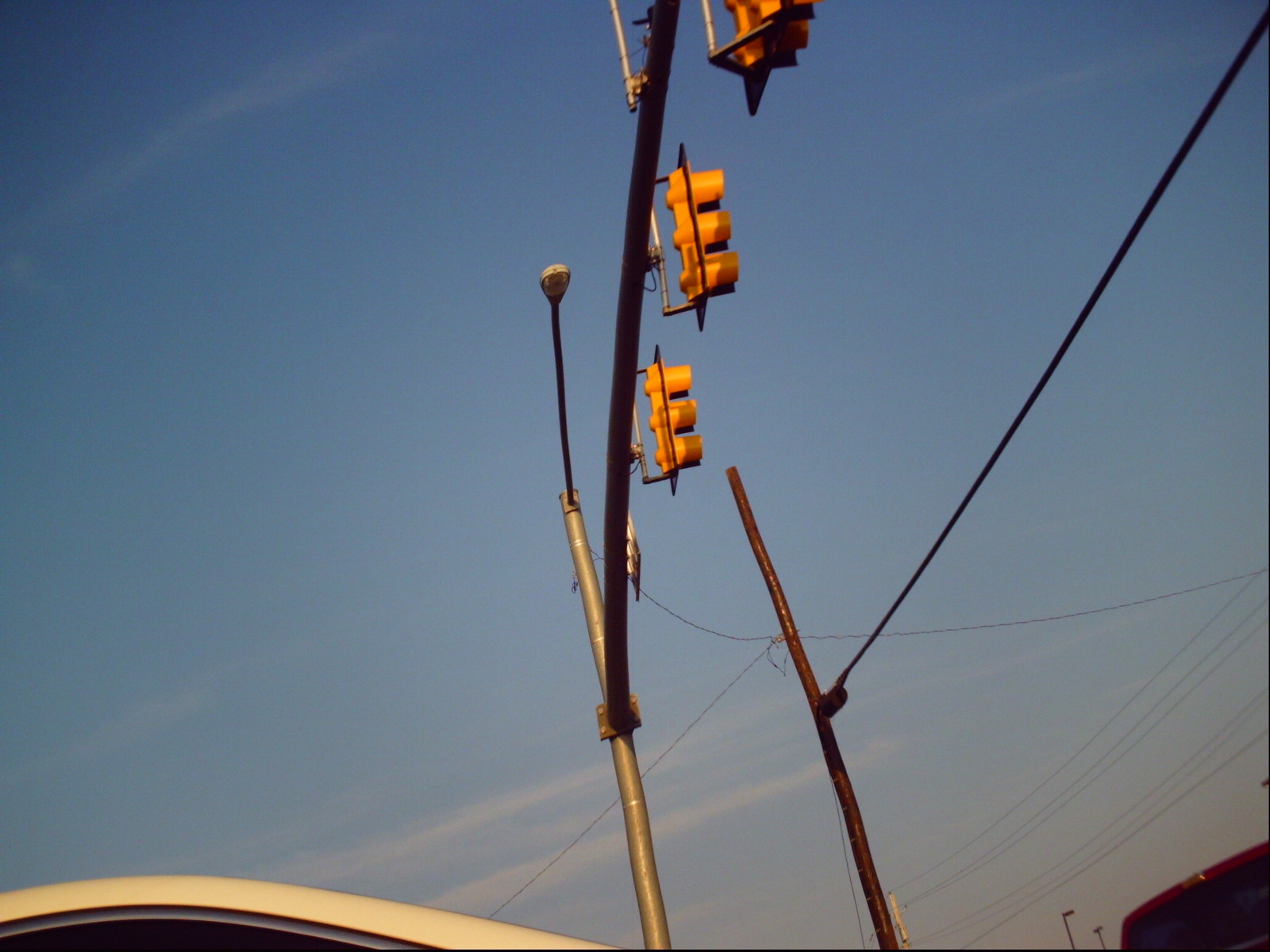In this photo, three vertically aligned stoplights are prominently displayed, though only two are clearly visible. These stoplights are mounted on a long, metal pole which extends upwards. The perspective of the photo is taken from ground level, looking up towards the stoplights. This pole is attached to a gray streetlight pole, from which an arm extends out, ending in a light bulb, indicative of a typical streetlight. Adjacent to this setup is a wooden utility pole with an attached electrical line. In the bottom portion of the image, part of a car's roof is also visible, providing a sense of scale and urban context to the scene.